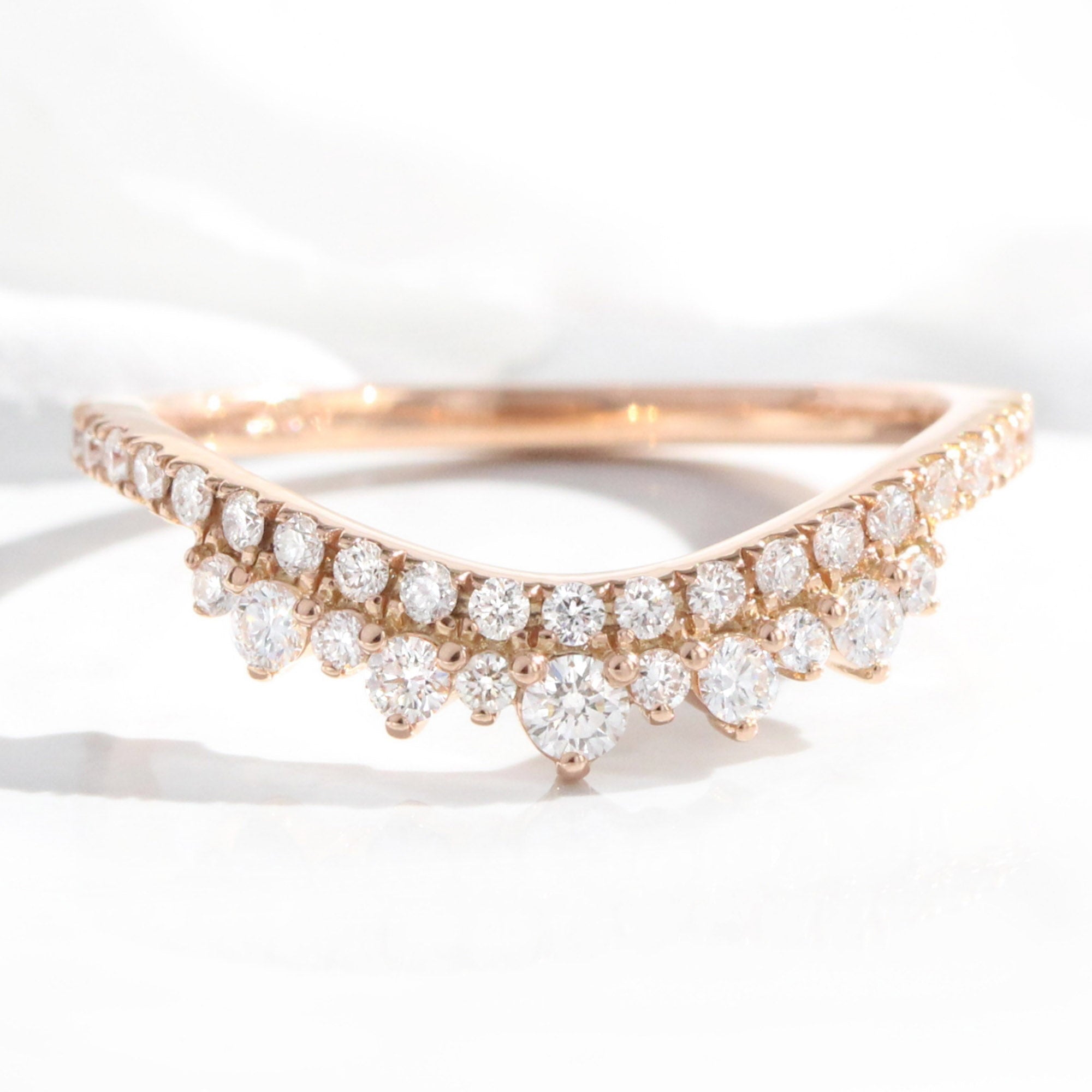This is a detailed photograph of a sophisticated piece of jewelry, likely a tiara or necklace due to its circular design with a slightly pointed front and sides. It features a stiff, rose gold base and is adorned with an intricate setting of round, bezel-set diamonds that cover most of its surface. The centerpiece displays a large diamond, flanked by alternating rows of small and larger diamonds, creating a lavish pattern that extends along the piece. The jewelry is placed on a white surface, casting a shadow beneath it, and the background is blurred, showcasing irregular bands of light blue. The close-up perspective makes the detailed craftsmanship appear larger, highlighting the exquisite arrangement of the diamonds.